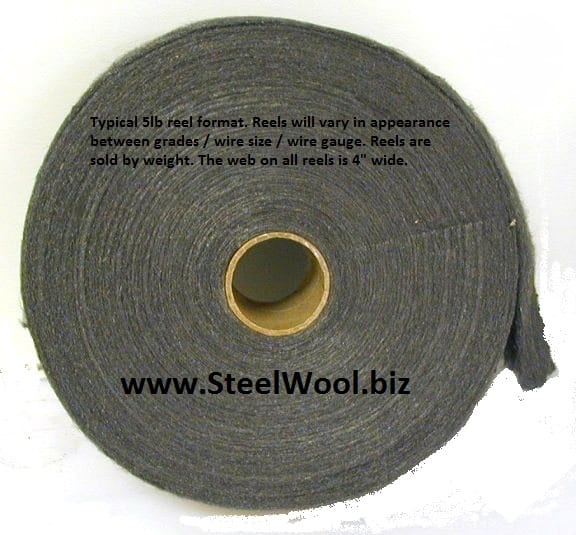The image is a detailed product photograph suitable for a sales website. It features a dark gray reel of gauze or fiber, centrally wound on a cardboard core, situated against a white background. A descriptive paragraph is overlaid at the top of the reel, detailing in black letters that it is a "Typical 5 pound reel format." The text specifies that reel appearances may vary depending on the grade, wire size, and wire gauge, and emphasizes that reels are sold by weight. Additionally, it informs that the web on all reels is 4 inches wide. At the bottom of the reel, the website www.steelwool.biz is also overlaid in black letters.